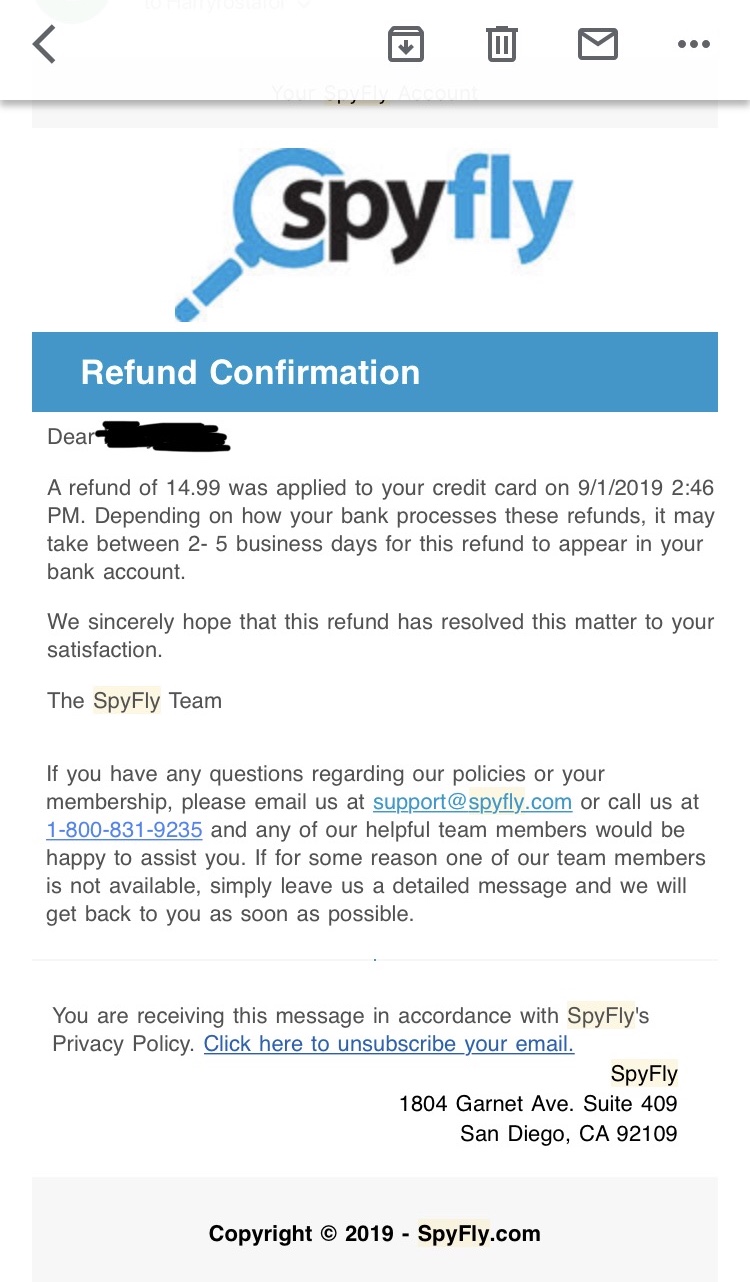The image is a screenshot of an email interface. At the top, a grey back button is visible alongside icons for saving (down arrow into a folder), deleting (trash icon), and marking as read/unread (envelope icon). Three vertical dots sit to the right of the envelope icon, suggesting more options. 

The primary content of the email is displayed against a white background with blue and black text. At the uppermost part of the email, there is a blue magnifying glass icon followed by the text "SpyFly," where "Spy" is colored black and "Fly" is blue. Beneath this, a blue banner with white text reads, "Refund Confirmation."

The main body of the email begins with "Dear [Name]," and goes on to inform the recipient that a refund of $14.99 has been applied to their credit card on September 1, 2019, at 2:46 PM. The email notes that the refund may take 2-5 business days to appear in the recipient's bank account, depending on their bank's processing times. 

Following this, the email expresses hope that the refund resolves the matter to the recipient's satisfaction and is signed by "the SpyFly team." Additionally, there is a prompt for further inquiries, providing both an email address, support@spyfly.com, and a phone number, 800-831-9235. The email reassures the recipient that any available team member will be happy to assist, or in the case they are unavailable, encourages leaving a detailed message for a callback.

Finally, there is a hyperlink at the bottom of the email for unsubscribing from future communications.